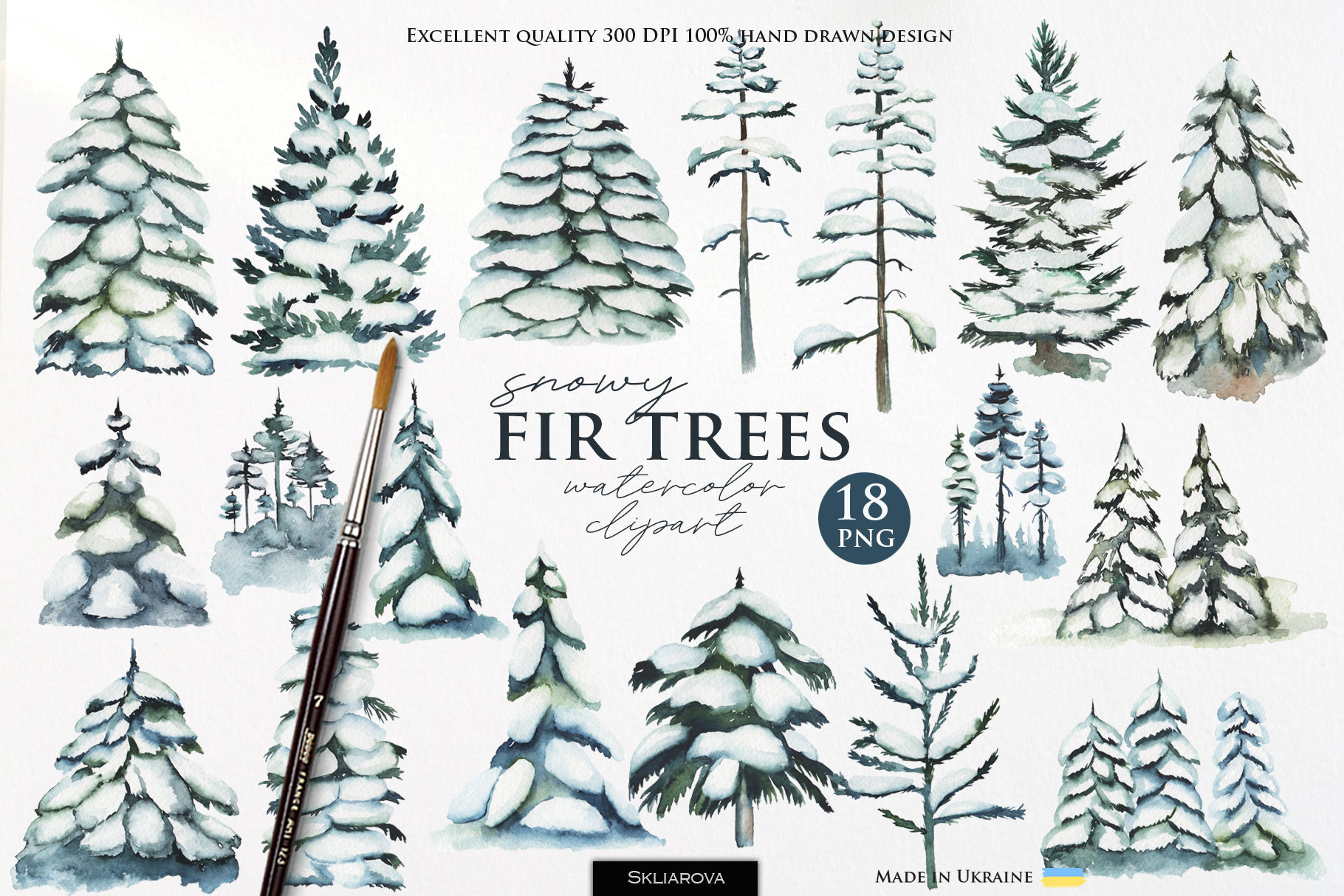This image appears to be an advertisement or a decorative item illustration for a set of watercolor clip art, featuring snowy fir trees. There are three rows displaying 18 different snow-covered fir tree designs, with some images containing multiple trees. The trees are illustrated in watercolor, indicating a hand-drawn quality emphasized by the text at the top which reads, "Excellent Quality, 300 DPI, 100% Hand-Drawn Design." In the center, it mentions "Snowy Fir Trees, Watercolor Clip Art" and "18 PNG" inside a green circle. The background is white, making the green trees stand out prominently. At the bottom, the word "SKLIAROVA" is displayed in a black rectangle, alongside a mark indicating "Made in Ukraine," accompanied by blue and yellow lines representing the Ukrainian flag. Laying across the left side of the image is a thin, number 7 watercolor brush, reinforcing the artistic nature of the product.